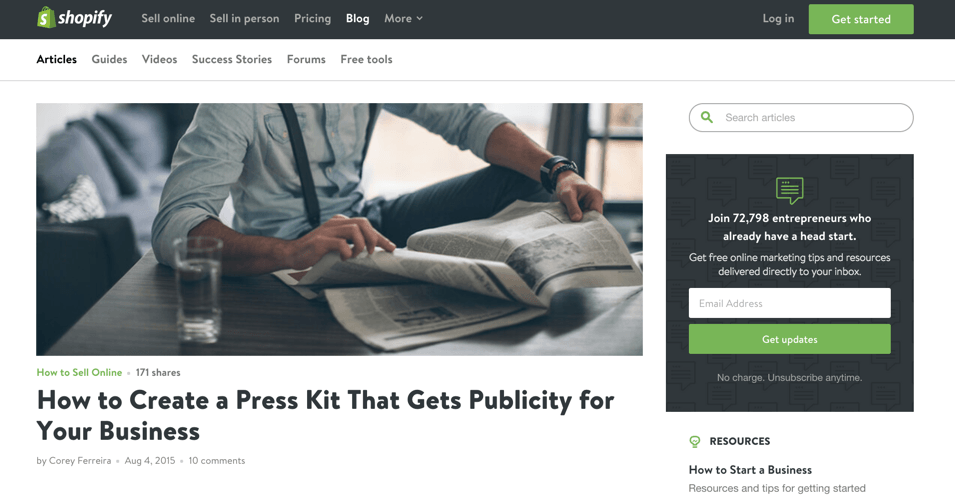In this image, the white background is adorned with various sections. At the top, there's a black header bar with a small green shopping bag icon featuring an "S" in the left corner, representing Shopify. Alongside it, the header reads "Shopify: Sell Online, Sell In Person," with options like "Pricing" and "Blog" highlighted. A dropdown menu titled "More" is visible next to the "Login" link, and a prominent green "Get Started" button is also present.

Below the header, on the white background, the content is organized into categories such as "Articles," "Guides," "Videos," "Success Stories," "Forums," and "Free Tools." This section is followed by a light blue divider line.

Central to the image is a photograph of a man reading a newspaper, accompanied by the headline "How to Create a Press Kit That Gets Publicity for Your Business."

On the right side, a search box is available for users to find specific content. Beneath the search box, another black box appears, featuring a green speech bubble icon at the top. This box prompts users to "Join 72,798 entrepreneurs who already have a head start," offering free online marketing tips and resources delivered directly to their inbox. There is a field for entering an email address and a green "Get Updates" button, with a note that there is no charge and the option to unsubscribe anytime.

At the bottom of the image, a small light bulb icon is displayed alongside the text "Resources," providing information on "How to Start a Business" and "Resources and Tips for Getting Started."